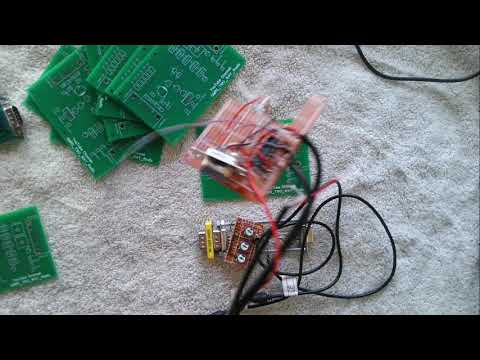This image showcases an assortment of electronic parts, primarily composed of seven green circuit boards with white markings, all laid out on a light gray towel. Positioned centrally and slightly right of center is an Arduino machine surrounded by a cluster of components. The Arduino features brown circuit boards and is nestled amid various wires, including prominent black, red, and green ones. Notably, a black wire with a white label can be observed in the upper right corner, although the text on the label is indiscernible. To the left of the circuit boards lies a male port end of a cord, embedded within the intricate setup of these parts. The scene hints at a potential computer assembly or electronic engineering project, with colors predominantly in green, white, black, and hints of silver, yellow, and pinkish hues. The image also suggests some motion blur, particularly around the central components, indicating possible movement during the capture.